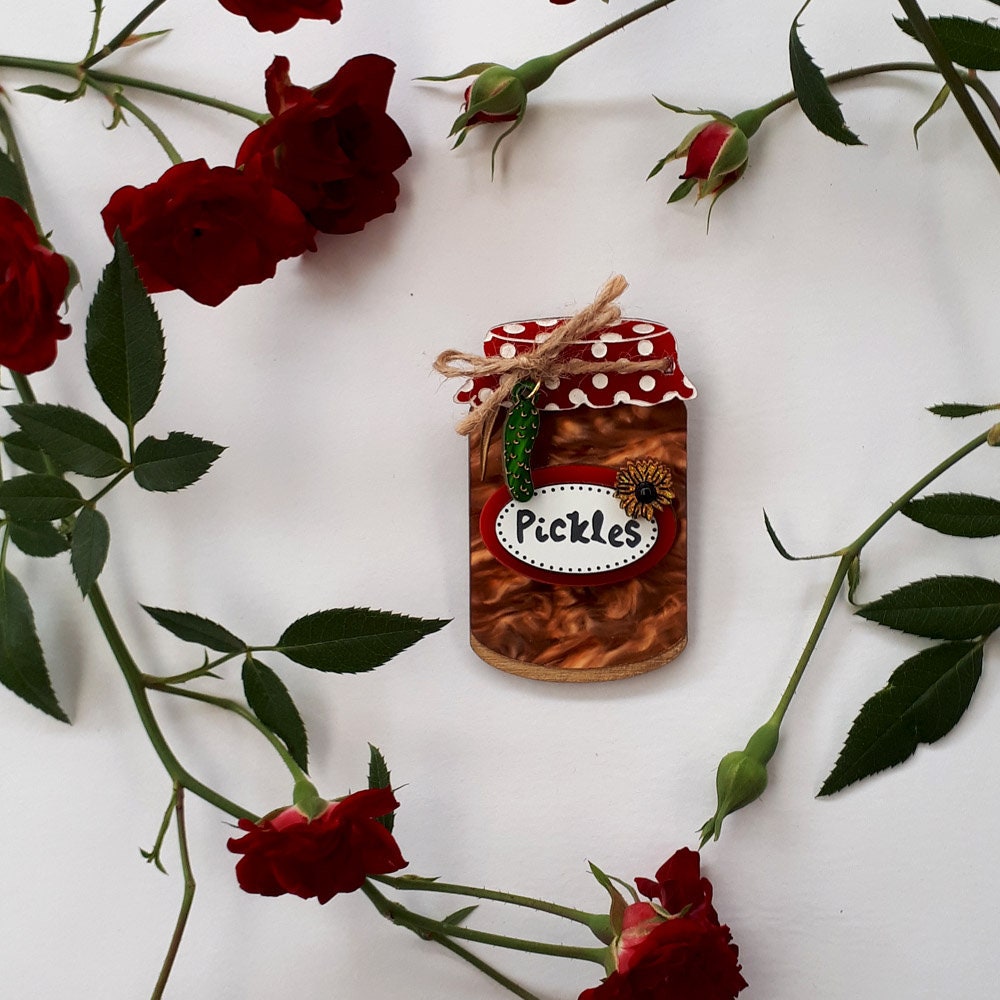This detailed photograph, possibly digital, captures a square image in an indoor setting illuminated by artificial light. The background is a light gray, providing a neutral canvas for the central element—a clear glass jar. The jar, which prominently features the word "Pickles" in black cursive on a label, is intricately detailed. The label is white, oval-shaped, adorned with black rim dots, and circled further by a red rim. A matching red and white polka-dotted lid tops the jar, secured with brown twine. Surrounding the jar, and casting delicate shadows on the background, are several cut red roses, laid from stems to blossoms. Some roses are fully opened while a few remain buds, adding a layered texture to the scene. Despite the label, the jar’s contents appear brown and do not resemble typical pickles, suggesting a different pickled item, possibly pickled beets. The overall composition, with its vivid contrasts and detailed elements, makes the photograph striking and thought-provoking.